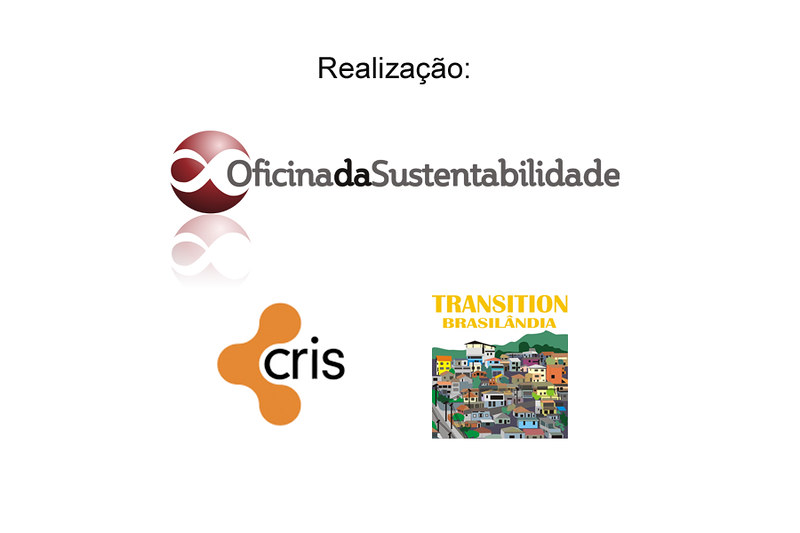The image is a detailed poster set against a white background, featuring several elements in a non-English language, which appears to be Portuguese. At the top, the word "REALIZAÇÃO" is written in bold black letters, with a squiggly line under the 'C' and above the 'A'. Below this, in dark gray letters, the phrase "OFICINA DA SUSTENTABILIDADE" is displayed next to a red circle containing a sideways white number 8. Underneath, on the left side, there is an orange logo made up of three connected circles, with the word "CRIS" inscribed in black lettering either inside or next to them. To the right of this logo, a colorful photograph depicts a town with numerous houses, streets, and a mountain in the background. Above this image, in yellow letters, the phrase "TRANSITION BRASILÂNDIA" is written, with an accent over the second 'A' in "BRASILÂNDIA".